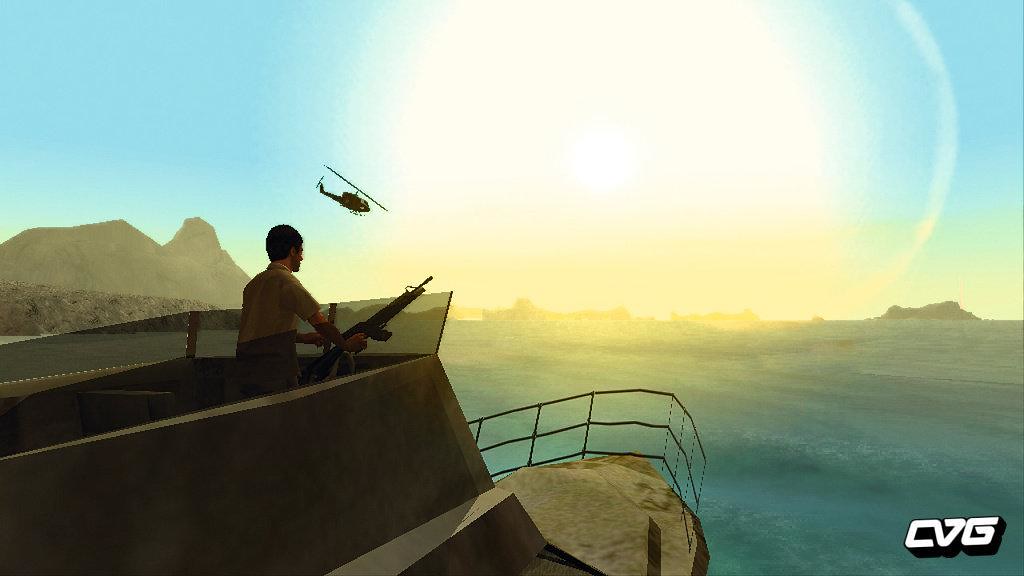This horizontally oriented color illustration, likely a screenshot from a video game, captures a dramatic and intense scene. At the bottom center, a boat with an architecturally unique, square-shaped top sails through a choppy sea. A man, standing on this rooftop, points a gun towards an intensely bright light or explosion near the horizon, slightly to the right of center. He faces away from the viewer, creating a sense of tension and anticipation. Silhouetted against the blinding light is a helicopter, flying directly into the luminous focal point of the scene. Surrounding the hull of the boat is a thin fence, highlighting the vessel's precarious situation. In the distance, rugged mountains frame the horizon line, adding depth to the dramatic seascape. The image is branded with the text "CVG" in white with a black border, located at the bottom right-hand side, suggesting it may be part of a series or promotion.